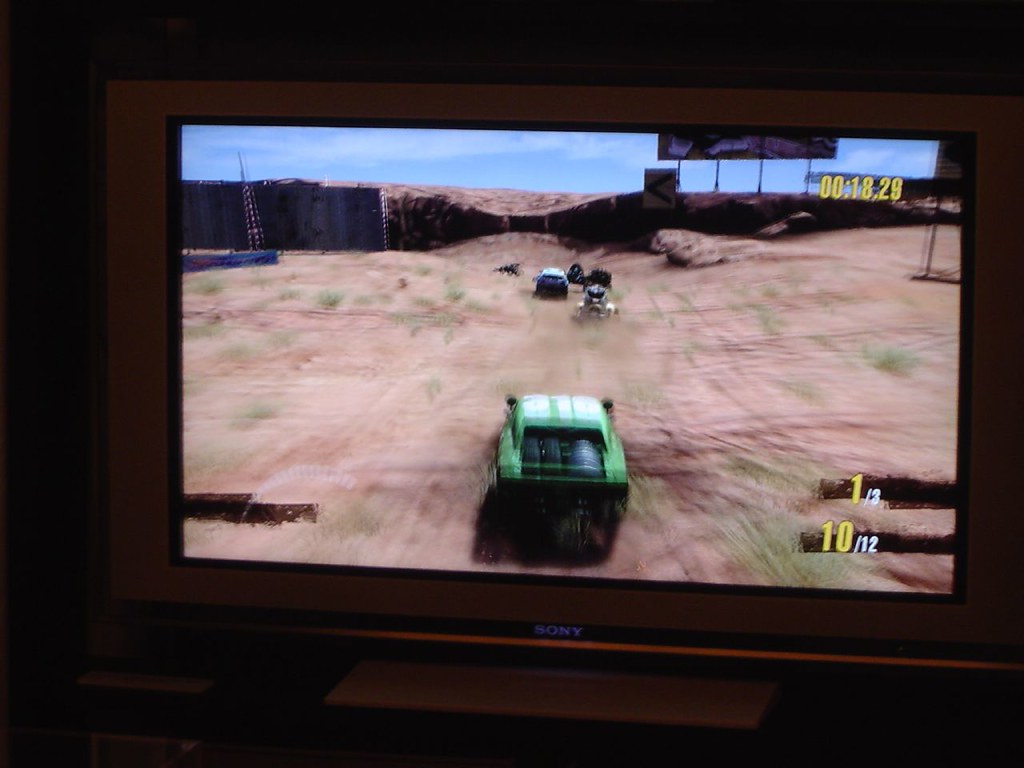In the dimly lit room, a photo captures a Sony television screen displaying a racing video game. The game features a green car, possibly numbered 315, which the player appears to be controlling as it races through a post-apocalyptic, sandy terrain with occasional minor green vegetation. The screen shows a time of 00:18.29 in the top right corner, alongside lap information at the bottom right indicating the player is on lap 1 out of 3 and currently positioned 10th out of 12 racers. The landscape features a broad, bumpy plain with a gradually narrowing road. Towards the right, a large billboard stands prominently, while to the left, a wall with a sizeable gap directs the cars' path. The image captures the intense, dusty scene with slight blurriness, emphasizing the dystopian setting and the competitive nature of the race.